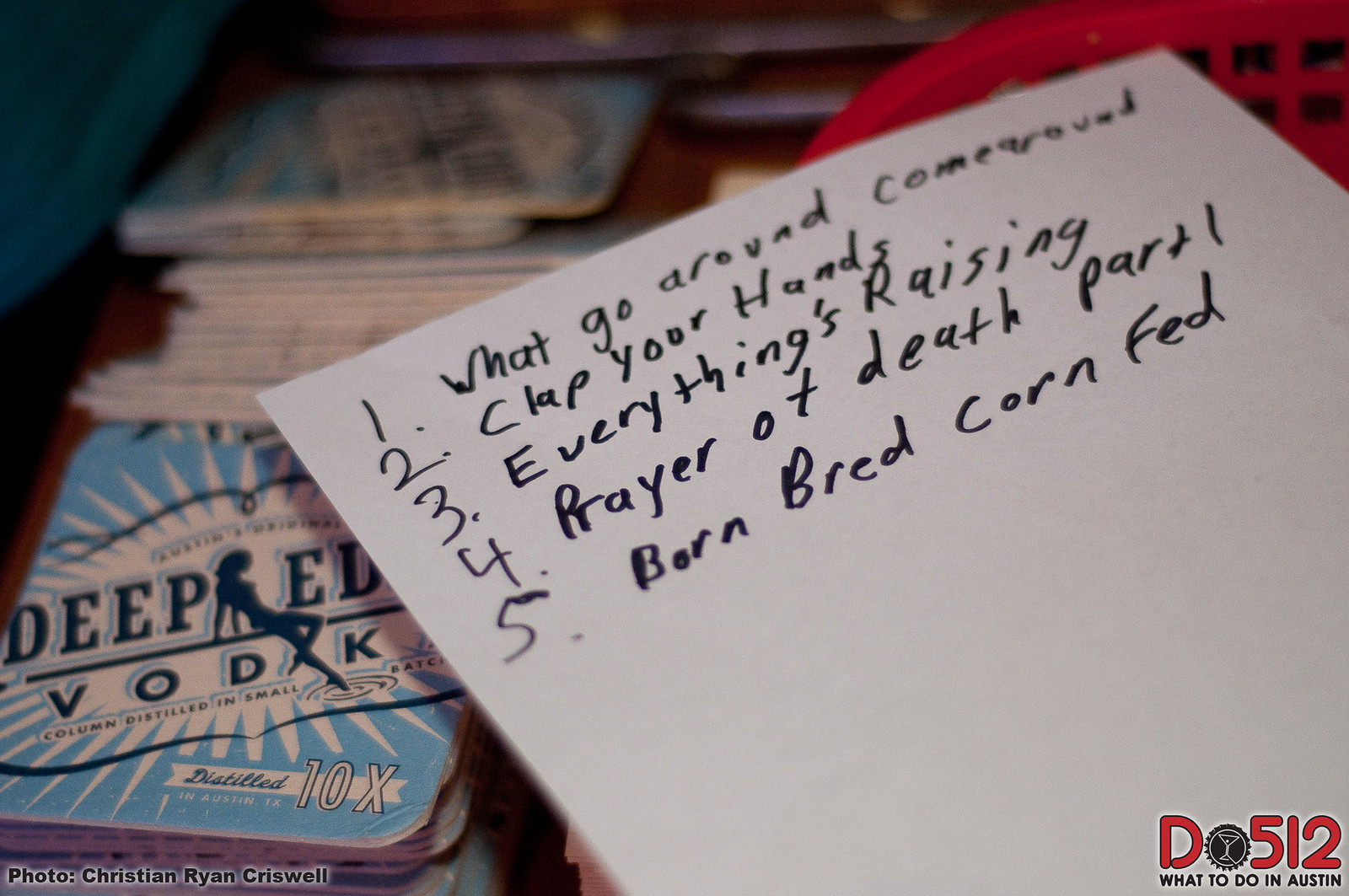The image is a color photograph in landscape orientation. The main subject is a white piece of notepaper tilted significantly to the left, laying on top of a stack of drink coasters. The notepaper, handwritten in black marker, lists five numbered items: 1. What goes around come around, 2. Clap your hands, 3. Everything's raining, 4. Prayer of death part 1, and 5. Born, bred, corn fed. In the bottom right corner of the paper, there is a circled "D" followed by the number "512" next to the text "What to do in Austin," featuring an "O" shaped like a gear. Under the notepaper, stacks of drink coasters are visible, mostly in blue and white, with designs including the words "Deep Eddy Vodka," "10x distilled," and a woman's silhouette sitting atop a black line. The coasters feature a white sunshine design against a blue background. The image is characterized by photographic realism, focusing on the notepaper and coasters, while the objects in the background remain mostly out of focus. In the bottom left corner, the photo credit reads "Photo: Christian Ryan Criswell."